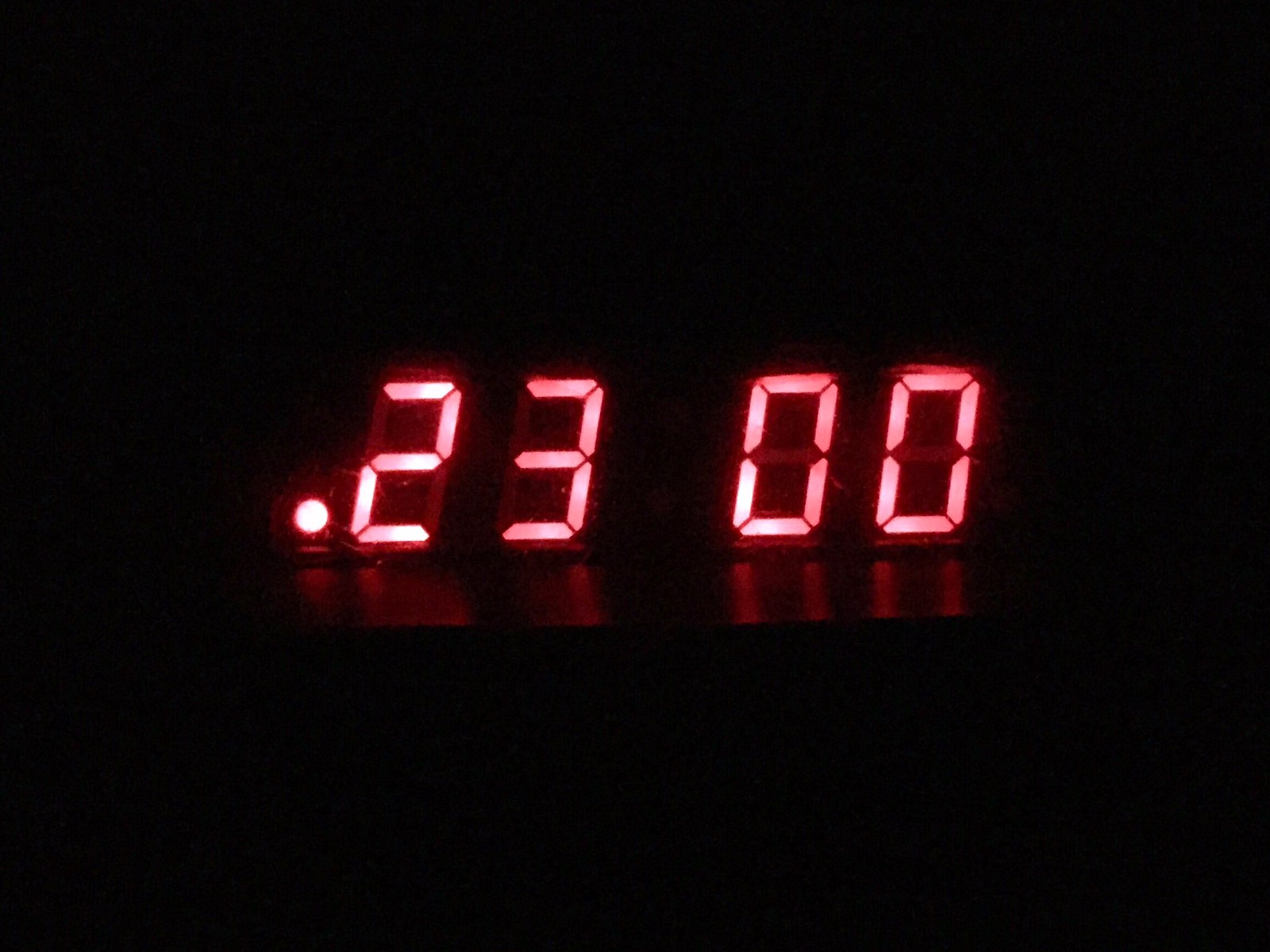The image depicts a digital readout of bright red numbers "2.300" on a completely black background. The display includes a dot followed by a 2, a 3, and then a space before two zeros. The 2 and the dot are particularly bright, while the 3 and the zeros are slightly less luminous. The red glow of the numbers is reflected on a hard surface below, indicating the device is placed on a table. Behind the illuminated numbers, the faint outlines of the unlit segments are visible. The overall setting is exceptionally dark, highlighting the vibrant red display as the focal point.